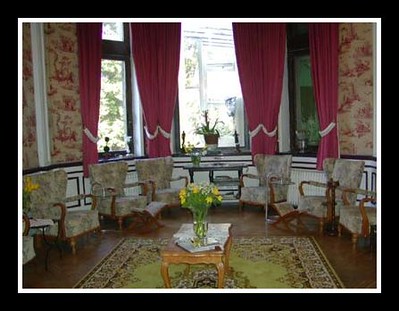The image captures a dignified living room with a circular layout, exuding a vintage luxurious ambiance reminiscent of a noble residence. Around the perimeter of the room are six wooden armchairs, three on each side, all featuring intricately embroidered upholstery. Between each set of three chairs, there is a small table. Centered in the bottom part of the image, a decorative rug hosts a square coffee table with elegantly curved legs, topped by a vase holding green and yellow daffodils. The room's upper section showcases a window adorned with dark red curtains, through which sunlight filters, illuminating a plant on the windowsill. The walls feature red and cream wallpaper with a white baseboard at the bottom, adding to the room’s refined aesthetic. The photograph itself is bordered by a white frame, encased within a thicker black border, hinting at a setting that could be a living area in a care home or a similar establishment.